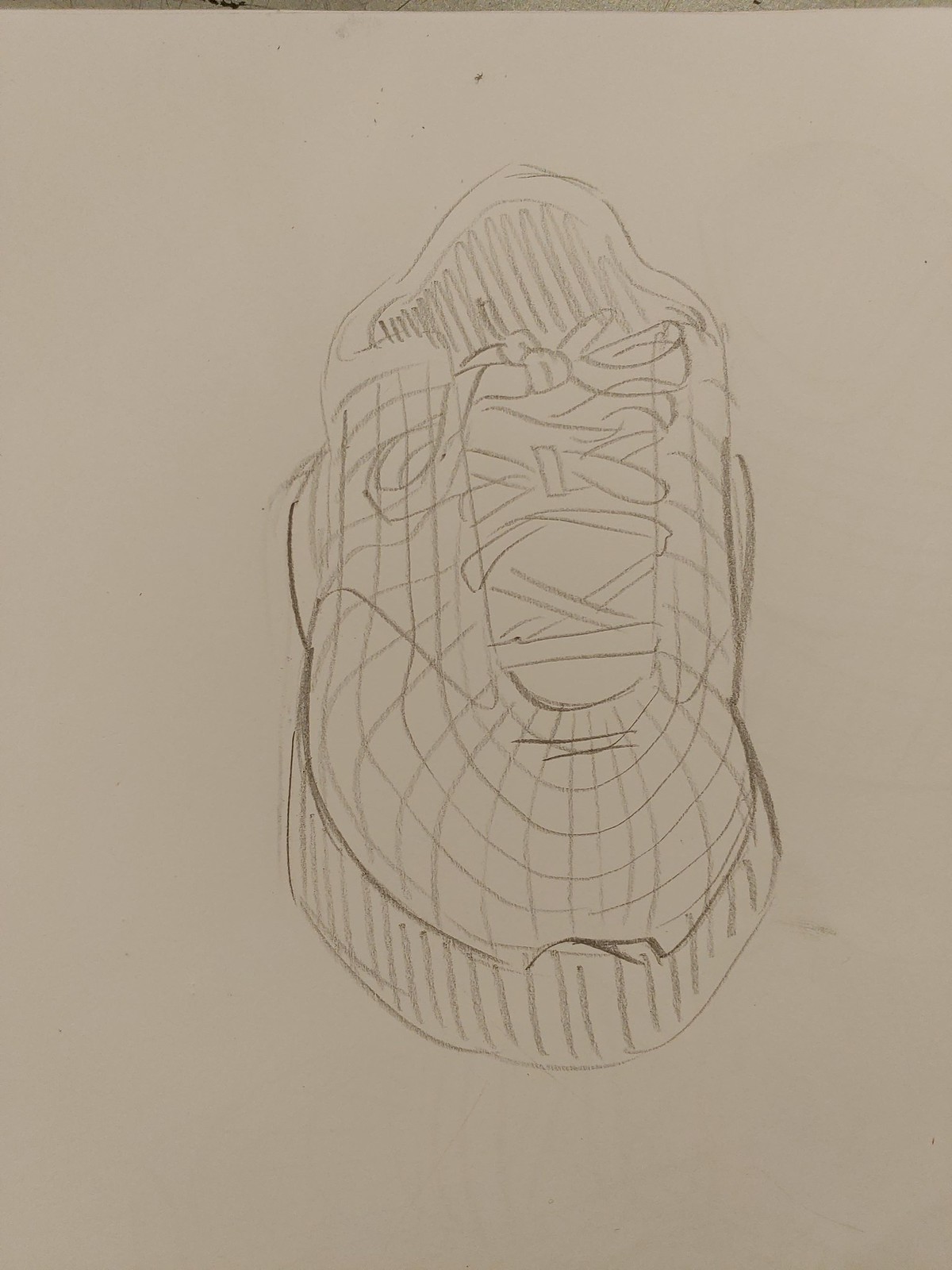This detailed black and white illustration is centered on a blank white sheet of paper, showcasing the front view of a shoe. Meticulously rendered in black ink, the drawing captures the intricacies of the shoe's design. The lower portion of the shoe features horizontal lines extending from left to right, suggesting texture or stitching. Above these lines, a series of concentric circles gradually decrease in size, adding depth and dimension to the shoe's form. The accurately depicted shoelaces are tied in a neat knot at the top, with the loose ends of the laces gracefully draping on either side. The simplicity of the white background highlights the meticulous craftsmanship and focus on detail in this monochromatic artwork.